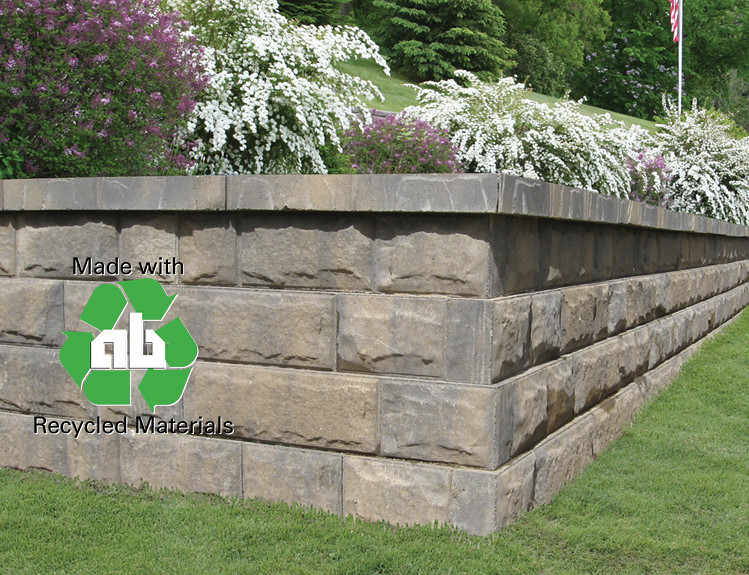The image features a landscaped outdoor area showcasing a rectangular, stone foundation crafted from recycled materials, as indicated by the inscription on the left side accompanied by three green, rotating arrows surrounding the letters "A" and "B." The structure, constructed with brownish-gray bricks, rises four layers high and serves as a ledge for a vibrant flower bed. This bed is adorned with bushes of purple and white flowers, enhancing the aesthetic appeal of the neatly manicured grassy surroundings. In the far background to the right, an American flag waves atop a flagpole, adding a patriotic touch. The backdrop is completed with an array of trees, including several pines, suggesting the setting is either in spring or summer within a clean, park-like area.